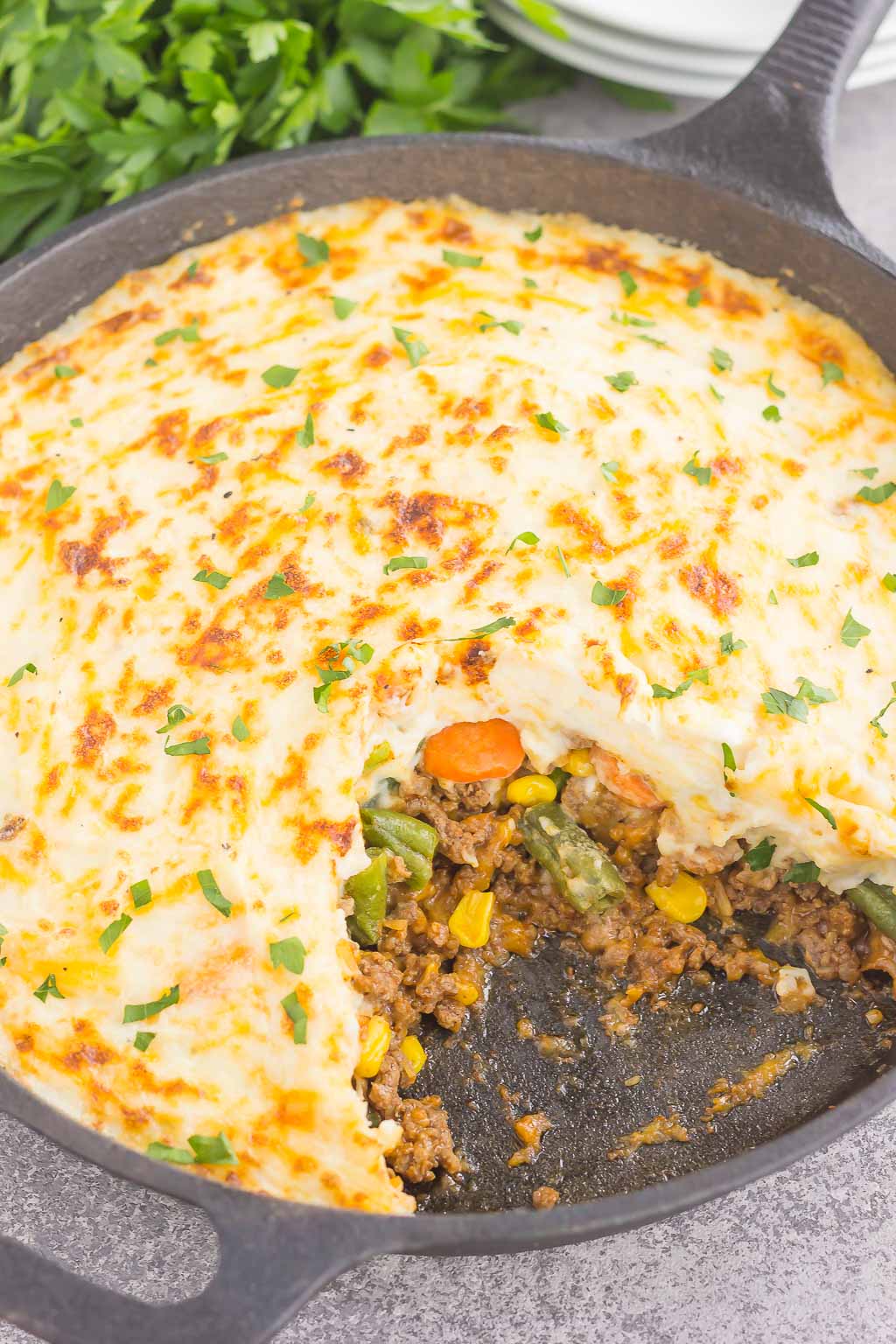A vibrant and hearty shepherd's pie is showcased in this photograph, captured in a large, circular cast-iron skillet. The skillet is positioned on a gray stone or countertop, adding a rustic outdoor ambiance to the scene. In the upper left corner, leafy green sprigs, possibly mint or other herbs, peek from the background, enhancing the earthy atmosphere.

The pie has a serving cut out at the far front, revealing its mouth-watering layers. The savory filling consists of browned ground beef mixed with green beans, carrots, and corn, all melded together in a rich, tomato-based sauce. This hearty mixture is generously topped with a layer of fluffy mashed potatoes, which have been oven-browned to a delightful golden hue, speckled with brown, giving a crisp texture to the top.

The finishing touch of finely chopped chives is sprinkled over the browned mashed potatoes, providing a pop of color and freshness. Off to the far right corner, only the edges of a stack of three white plates are visible, subtly indicating readiness for serving. This beautifully browned and garnished shepherd's pie promises a comforting and delicious meal.